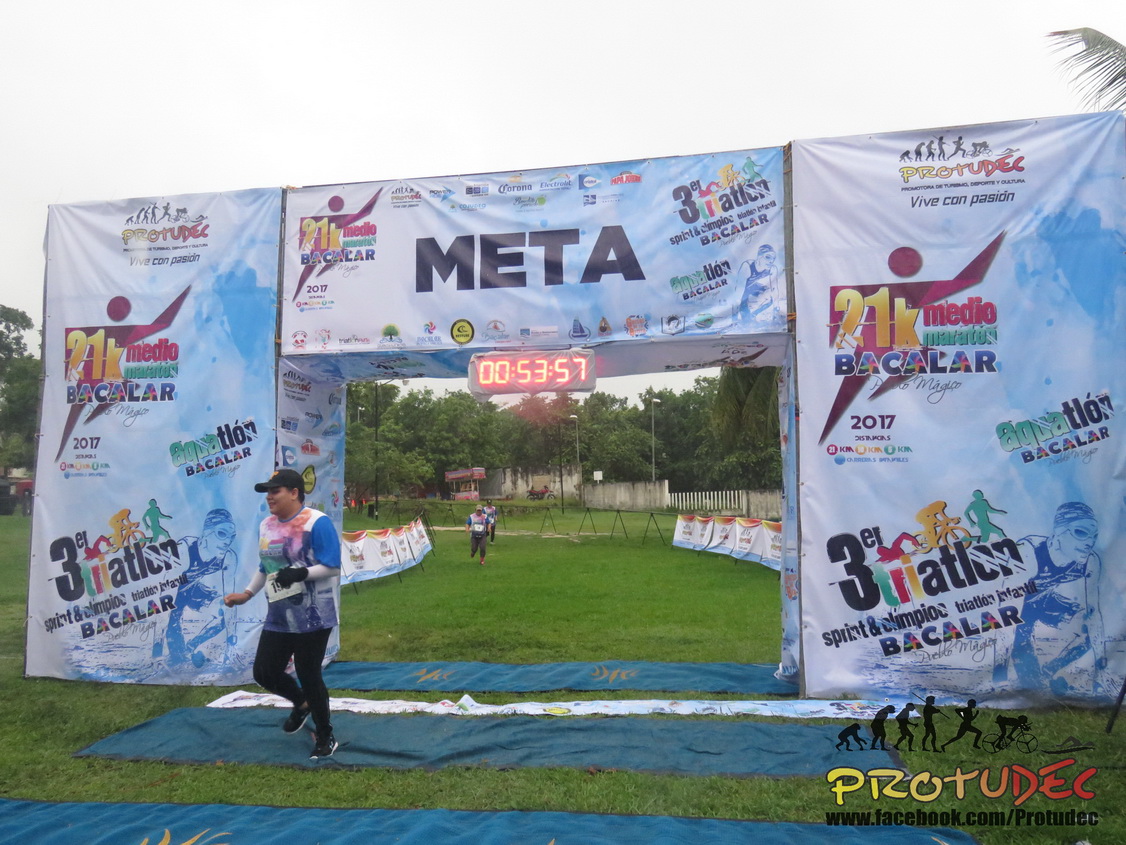The image captures the finish line of a grass-based racing track, presumably for a triathlon event, adorned with a light blue canopy. Prominently, "meta" is displayed at the top of the canopy. The finish line structure consists of two pillars connected by a horizontal framework featuring red digital numbers that read "005357". Various advertisements decorate both sides of the canopy, showcasing local sponsors and promotional material. A detailed illustration on the right-side canvas depicts the evolution from a monkey to a human, then transitioning to a runner, cyclist, and swimmer, encapsulating the essence of a triathlon. A man, in a blue shirt and cap, has just crossed the finish line, with another runner visible in the distance. The setup includes all elements found in a professional race scene, emphasizing the completion of the event.